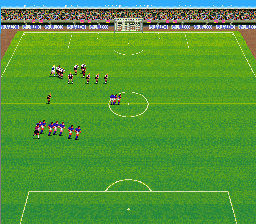A detailed, cleaned-up caption would be:

An AI-generated image presents an angled aerial view of a vibrant soccer field. The field is a medium chartreuse green, featuring large white rectangles at either end, denoting the goal areas. At the far end of the field, a visible goal structure stands, accompanied by packed bleachers filled with indistinct spectators, set against a clear blue sky. A distinct center line and circle are prominently displayed in the middle, within which three players can be spotted. At the forefront of the image, we see seven players donning blue shirts and red shorts, possibly accompanied by a coach walking alongside them. Across the center line, there are nine more individuals, potentially a mix of players and officials. The scene is bustling with activity, capturing the essence of a lively soccer match setup.